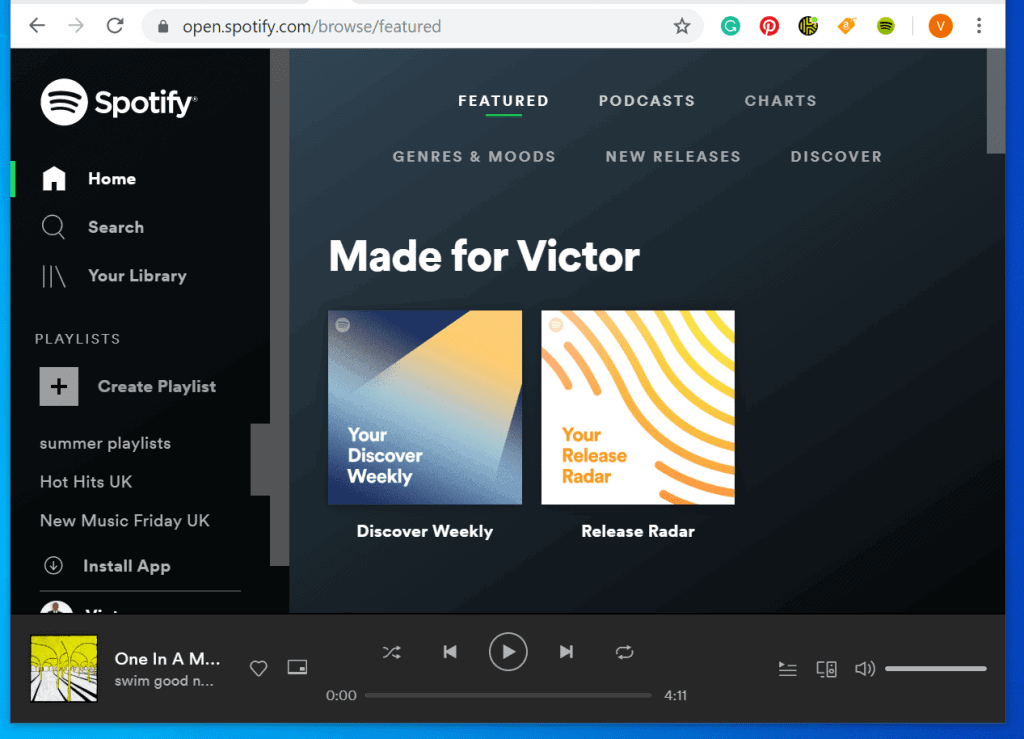This online image showcases the Spotify website interface. At the very top of the page, there's a banner featuring a search bar. Inside the search bar is a lock icon and the URL "open.spotify.com/browse/feature". There is a star icon on the right side of the search bar, which, when clicked, saves the page to your bookmarks. 

To the right of the search bar, there are several icons, including a green tab to reload the page, a Pinterest icon, and various other icons. Additionally, there is an orange profile circle with the letter "V" in it.

On the left-hand side of the page, the Spotify brand logo is prominently displayed. Below the logo, there is a vertical navigation menu. The first item is a home icon labeled "Home." Following that are a search icon and the label "Your Library." Next, there's an option for "Playlists," accompanied by a white square with a black plus sign, allowing users to create a new playlist. Further down the menu, there are labeled playlists: "Summer Playlist," "Hot Hits UK," and "New Music Friday UK." At the very bottom, there is an "Install App" option, signified by a circle with a downward arrow, providing the functionality to install the Spotify app.